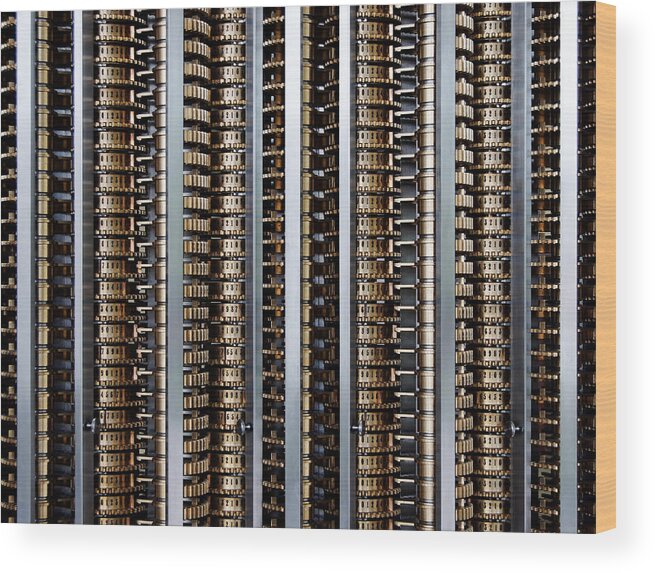The image captures an extreme close-up of a highly symmetrical arrangement of gears, possibly part of a paper shredding or document destroying machine. The gears, bronze or whitish gold in color, are meticulously aligned in rows and columns, creating a visually striking and intricate pattern. In between the gears, there are long gray steel beams, some of which feature bolts or nuts. Each gear has sharp indentations and indented black numbers, adding to the machine-like appearance. The overall color scheme includes shades of gold, brown, and gray, and the design is so precise that it evokes the appearance of a mechanical structure or even a side view of skyscraper balconies. The entire setup is contained within a square frame, displaying about 14 vertical rows of these repeating gears and beams.